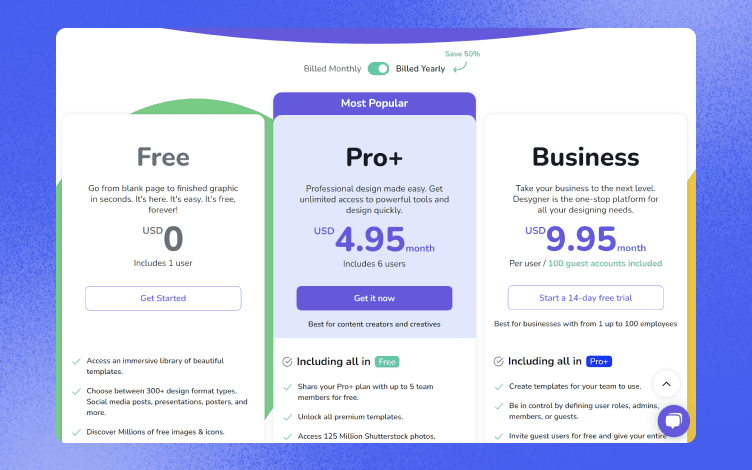This image showcases a website's subscription plans, framed by a border combining dark purple, light violet, and white colors. Inside, the primary background is white. At the top center, there is a purple border; at the bottom left, a green border; and at the bottom right, a yellow border. The subscription plans are presented in three tiers:

1. **Free Tier**: Located on the left side, this plan includes one user. At the bottom, there is a "Get Started" button.
 
2. **Pro Plus Tier**: Positioned in the center, this is the most popular plan, priced at $4.95 per month. It includes six users and features a "Get It Now" button below it.

3. **Business Tier**: On the right side, this plan costs $9.95 per month and offers a free 14-day trial, indicated by a corresponding button.

At the top, an option to toggle billing periods is displayed, with the switch currently set to "Build Yearly - Save 50%".